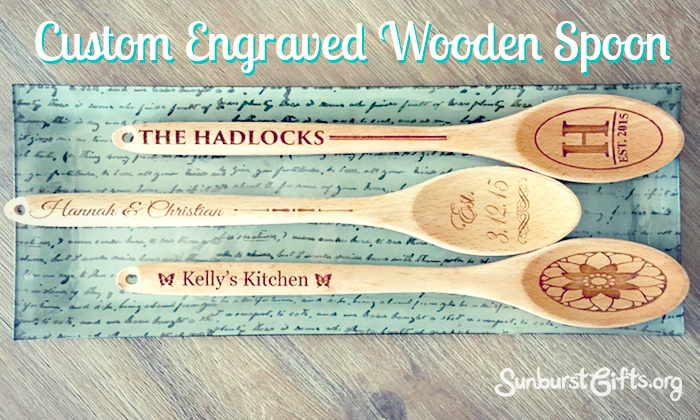The advertisement features three intricately custom-engraved wooden spoons displayed on a light mint green rectangular tray with cursive writing on its surface. At the top of the image, a banner reads "CUSTOM ENGRAVED WOODEN SPOON," while the URL sunburstgifts.org is seen in the lower right corner. 

Each spoon showcases unique details: 

- The top spoon has "the HADLOCKS" engraved on the handle, with a large, serif-font "H" and "EST. 2015" etched on the flared portion.
- The middle spoon reads "HANNAH & CHRISTIAN" in cursive on the handle, accompanied by "EST. 3.12.15" on the spoon part.
- The bottom spoon displays "KELLY'S KITCHEN" in a Garmond font on the handle, framed by two butterflies on either side, and a flower design on the spoon's wide part.

The composition highlights the fine craftsmanship and personalized nature of the product, emphasizing its appeal as a thoughtful and unique gift.